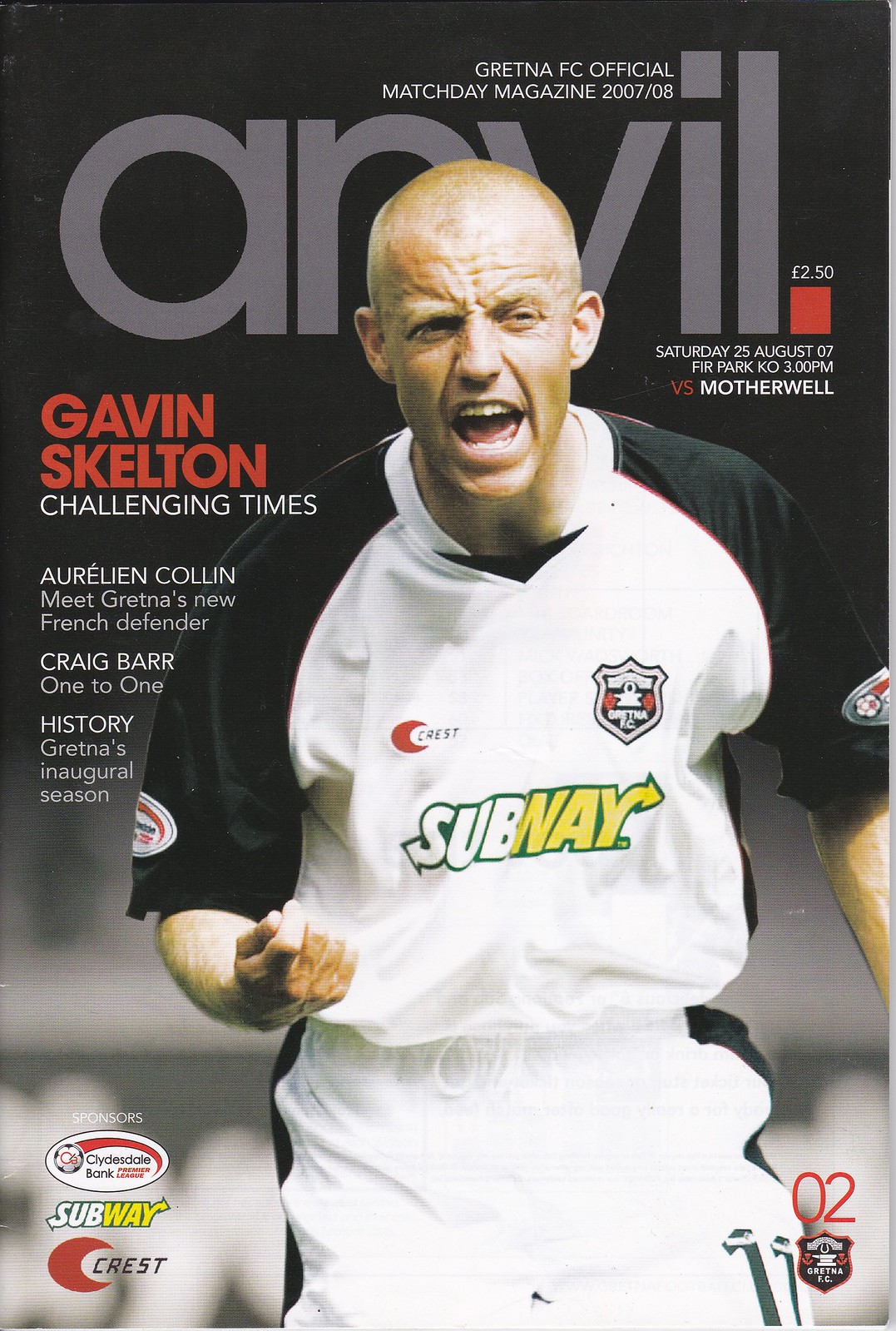This image portrays the cover of the "Gretna FC Official Match Day Magazine" for the 2007-08 season, featuring a football-themed design. Dominated by a dark, blurry background which transitions into visible sponsor signs of a football pitch, the cover prominently showcases a male footballer in a white shirt with black sleeves—also adorned with a Subway sponsor's logo. The player, identified as Gavin Skelton, wears jersey number 11 and is captured in an emotional moment, either yelling or grimacing, with a closely-cropped haircut or possibly bald.

At the top, the magazine title “Anvil” is displayed in large gray letters, partially obscured by Skelton's head, with the subtitle "Gretna FC Official Match Day Magazine 2007-08" in smaller white font. A red square displaying the price "£2.50" and the match details "Saturday 25 August 07, FR Park, KO 3 p.m., vs. Motherwell" is also visible.

Additional text around the cover includes phrases like “Gavin Skelton: Challenging Times” in red font to the left of him, and other features such as "Arlene Cullen: Meet Gretna's New French Defender" and "Craig Barr One-to-One: History, Gretna's Inaugural Season" in white font. The lower portion of the cover includes more sponsor logos, such as Subway and Crest, with an "o2" logo and a shield symbol on the right side.